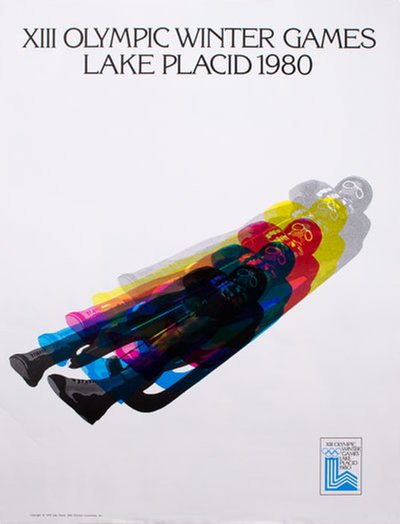This image is a promotional poster for the XIII Olympic Winter Games held in Lake Placid in 1980. The background is a grey color, providing a neutral backdrop to the vibrant elements of the design. At the top, the headline prominently displays "XIII Olympic Winter Games, Lake Placid 1980" in black letters. The central graphic features a person engaging in the sport of luge, depicted as reclining back in a sled. The image is creatively superimposed in multiple, vibrant colors—black, blue, red, yellow, and grey—giving the impression of motion as the person slides diagonally, from the bottom left to the top right. This color layering creates a dynamic aura around the figure. At the bottom left corner, there's an unreadable footnote in small text. The bottom right corner includes the official logo of the 1980 Lake Placid Olympic Games, characterized by its blue and white spiral design and the Olympic rings. Despite some obscured text, the overall composition vividly evokes the energetic and competitive spirit of the Winter Games.